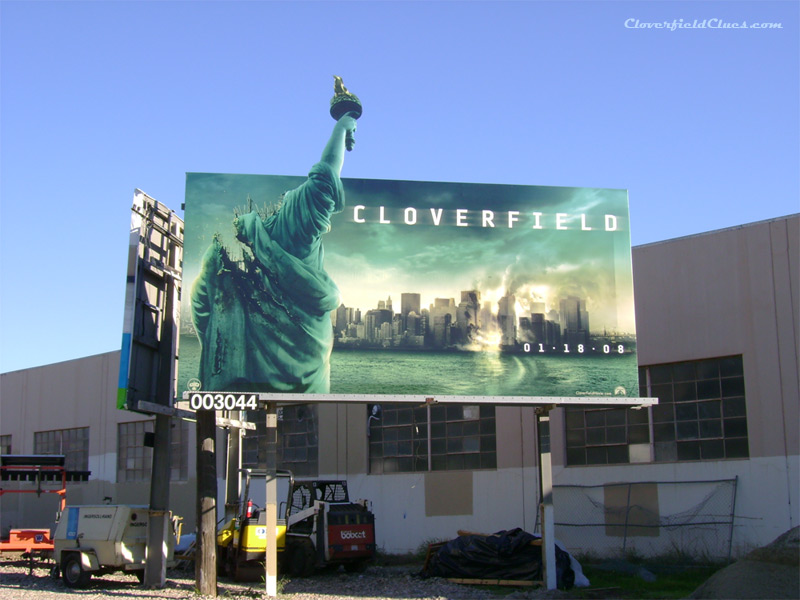The image shows a large billboard advertisement for the movie "Cloverfield" in front of a two-tone industrial building. The building backdrop features white and brown sections with various square windows. The billboard, mounted on two grey poles, prominently displays a chaotic city skyline at sunset, with smoke rising from buildings across a river. The main focus is a dramatic image of the Statue of Liberty viewed from behind; her head is missing, and her raised arm with the torch extends beyond the top edge of the billboard. The movie title "Cloverfield" is written in white text on the blue background of the billboard. Below, the date "01.18.08" is displayed near the waterline. Additionally, at the bottom left corner of the billboard, the number "003044" is printed in white on a black background. There are also several construction vehicles, including a Bobcat and a yellow and black machine with a red fire extinguisher, positioned below the billboard. Another billboard in the background faces away from the viewer, adding to the industrial ambiance of the scene.